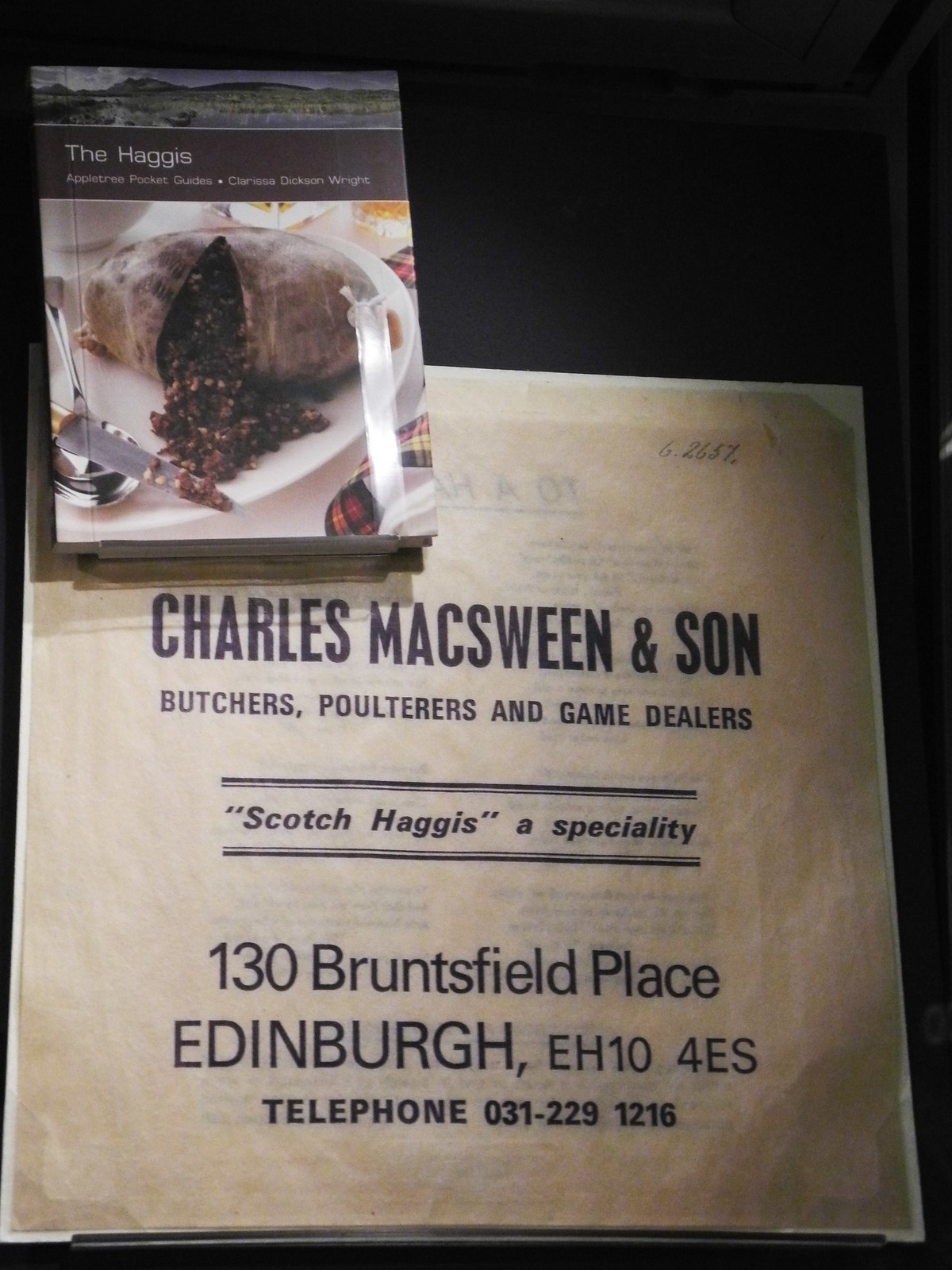The image showcases a vintage advertisement sealed in a protective covering, set against a plain off-white background with black text. The advertisement is from "Charles McSween and Son," identifying them as butchers, poulterers, and game dealers. It highlights "Scotch Haggis" as a specialty. The detailed address provided is 130 Bruntsfield Place, Edinburgh, EH104ES, with a telephone number of 031 229 1216. In the top left corner of the frame, there's a book titled "The Haggis Apple Tree Pocket Guides" by Clarissa Dixon White, suggestive of a haggis cookbook. The advertisement appears very old and yellowed, adding to the nostalgic appeal of the image.